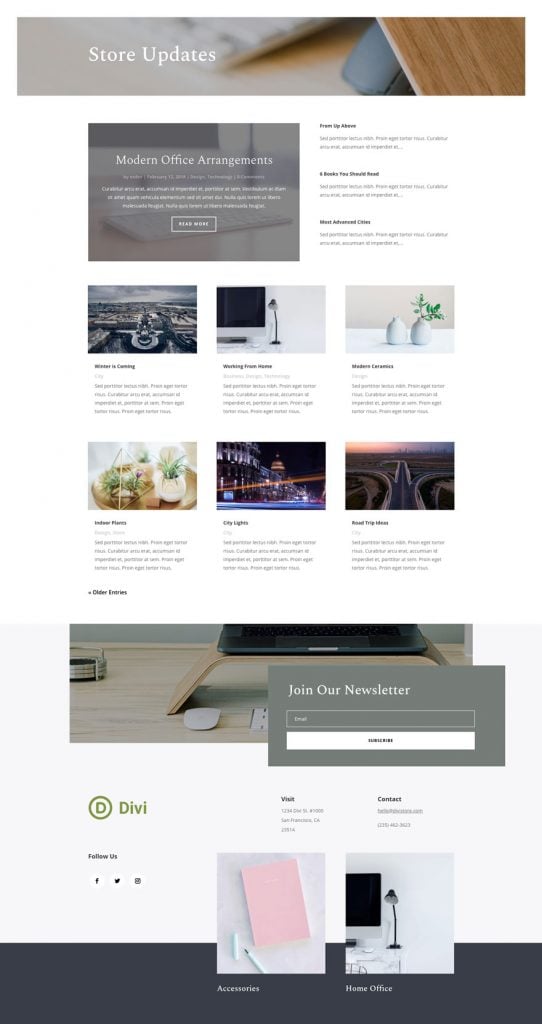This image is a detailed screenshot of an online store focused on office design and organization.

At the very top, the header reads "Store Updates," followed by a prominent photo, likely depicting a desk setup. Beneath this image, the background is stark white with a noticeable gap. Underneath this gap, there's a grayscale banner titled "Modern Office Arrangements," accompanied by an unreadable wall of text consisting of several paragraphs.

On the right side of this section, there's a small menu-like structure featuring three bullet points, each paired with a brief paragraph or sentence of text. Further down, there is roughly an inch of white space before two rows of images. Each row contains three photos, making a total of six images. Below each image, there are bolded two to three-word descriptions, followed by one to two descriptive sentences providing an overview or general details about the business.

Continuing down, there is another photo of a desk complete with organizing materials. Adjacent to this image, a call-to-action section invites users to "Join Our Newsletter," featuring a grayed-out box where users can enter their email addresses and a white box labeled "Subscribe."

At the bottom-left corner, there is a logo—a 'D' inside a circle with the letters "DV"—followed by a navigational menu on the right. Finally, at the very bottom of the page are two more images labeled "Accessories" and "Home Office," reinforcing the theme of office design and organization.

Overall, this screenshot is from an online store dedicated to providing solutions for organizing and designing home or work office spaces.